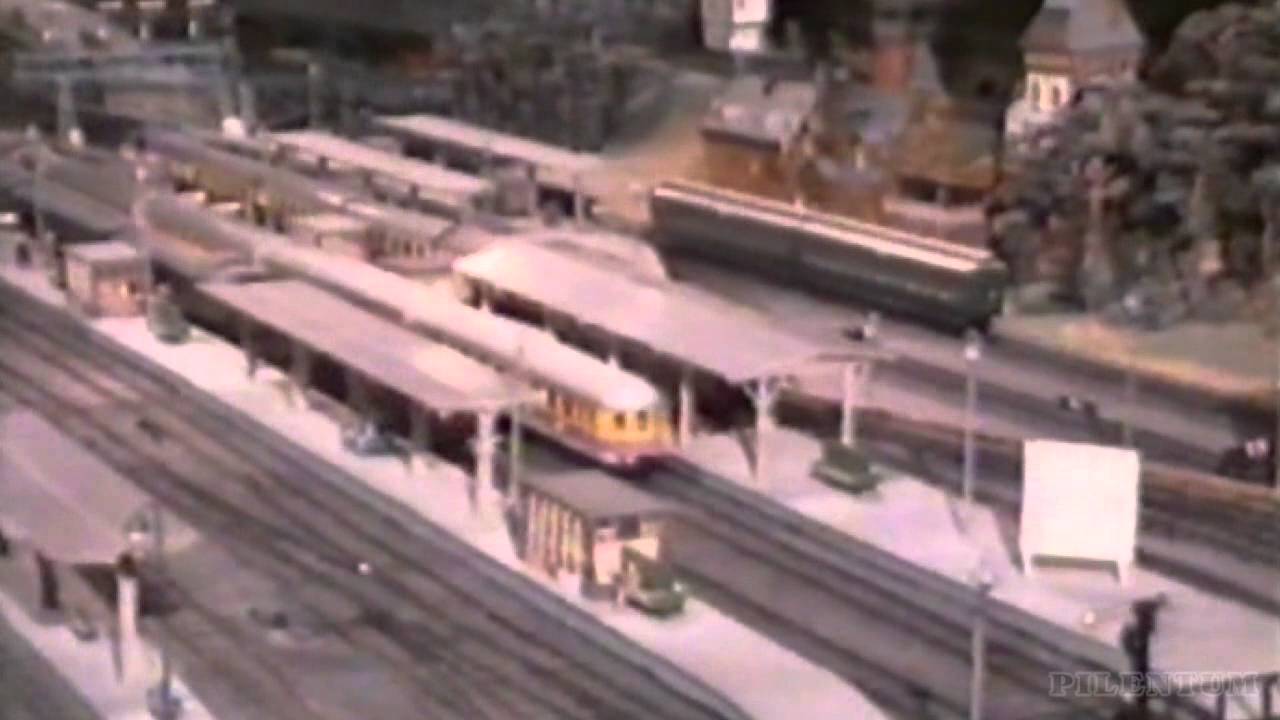This detailed photograph, though blurred and seemingly old, captures a model train station scene. The centerpiece of the image is a miniature train station with multiple tracks, up to four, each featuring different arrangements. Central to the layout is a long yellow train with a white top, positioned on the second track, while the fourth track hosts a large, silver two-car train. The first and third tracks appear empty. The station platform includes benches and a covered area. Surrounding the tracks are various miniature buildings, predominantly brown, complemented by greenery and trees that frame the scene. Scattered throughout the station are various signs, adding to the intricate detailing. The muted colors of greys, greens, and browns dominate the image, with the bright yellow train standing out distinctly.